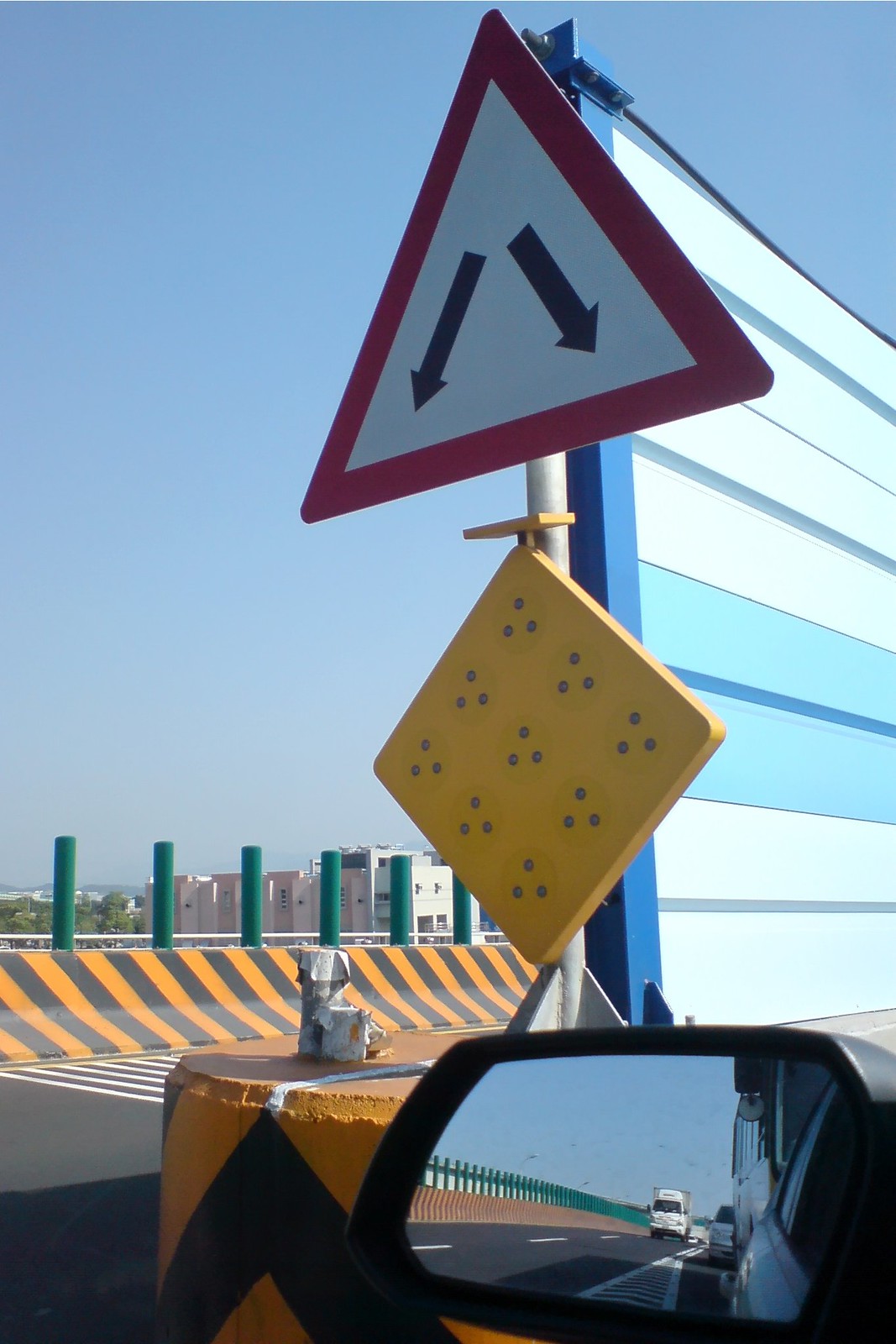In the foreground, at the bottom right corner of the photo, a side view mirror of a car driving on the right side of the road is visible, reflecting some traffic behind. Oncoming traffic is led by a large white transport vehicle on the opposite side of the road. Central to the photograph is a prominent road divider topped with dual warning signs. One sign is a yellow diamond and the other is a white triangle with a red border, featuring arrows pointing left and right to indicate permissible driving sides around the divider. The base of this divider is marked in yellow with bold black zigzag patterns, alerting drivers to its presence.

The divider itself is constructed from strips of opaque white and blue metal, forming a solid barrier that prevents drivers from seeing the lanes on the opposite side. Background details include a concrete barrier painted with yellow and black diagonal stripes, alongside green pylons stationed atop the barrier, running parallel to the divider. The car’s rearview mirror offers a glimpse of this pattern extending down the road, demonstrating the continuity of the roadway's edge as far as the eye can see.